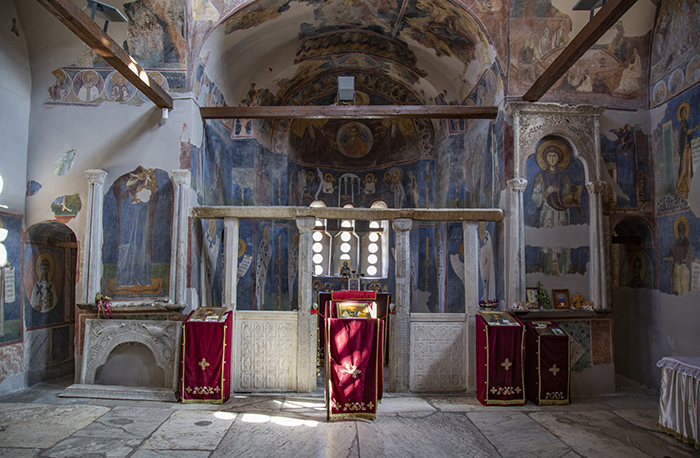This detailed photograph captures the interior of a historic European church with multiple intricate architectural and artistic elements. The flooring is paved with slate and white marble, and it appears that some figures have been buried beneath the slate, a common practice in ancient churches. The walls are pale blue and adorned with numerous religious icon paintings set against a blue background. Dark wood beams stretch from the front to the back, supporting the structure, and there's an arched ceiling above the nave area.

In the foreground, four podiums are draped in rich burgundy cloth with golden decorations, including embroidered crosses, suggesting a Christian affiliation. These podiums, two on the right, one in the center, and another slightly to the left, stand prominently. Beyond them, there is a fireplace area with arched religious paintings above, depicting various biblical scenes and figures.

The back walls are white and adorned with religious murals, and more paintings grace the ceiling, contributing to the sacred atmosphere. The overall ambiance and design elements, including the cloth-covered altars and murals, emphasize the church's historical and religious significance.